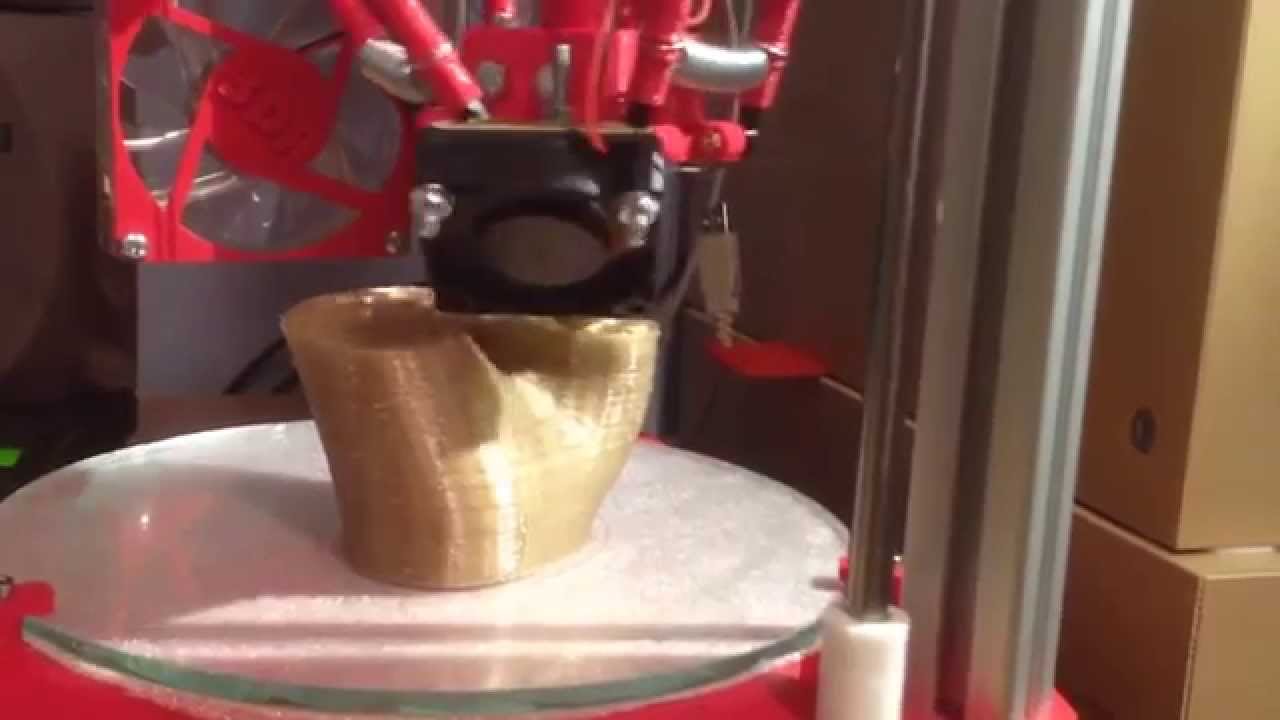The photograph depicts a detailed, albeit slightly blurred, scene of a mechanized setup potentially involving a 3D printing process. Central to the image is a gold-colored object with a textured, abstract design, resembling a curvaceous vase. This object is being created by a red and black 3D printer. The 3D printer features a clear, round plexiglass plate on top, and extends grey metal rods upwards. The setting seems industrial or workshop-like, evident from the scattered brown cardboard boxes on the far right side. Additional elements like bolts, nuts, and joints hint at the mechanical complexity involved. The image is characterized by a variety of colors including red, silver, white, black, brown, and gold, and the indoor environment is suggested by the lighting and shadows present.